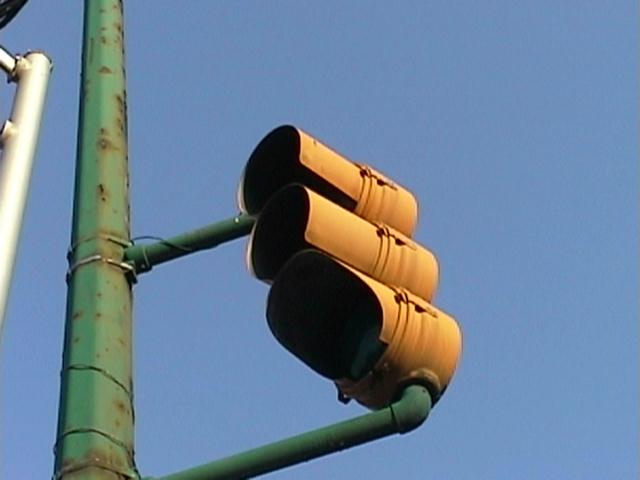A close-up, upward-facing view of a yellow traffic stoplight, mounted on two poles that converge into a larger structure. The image captures the left side profile of the stoplight against a clear blue sky, obscuring the actual traffic lights (red, yellow, and green) inside. The bright yellow color of the stoplight stands out prominently, contrasting sharply with the vivid background.